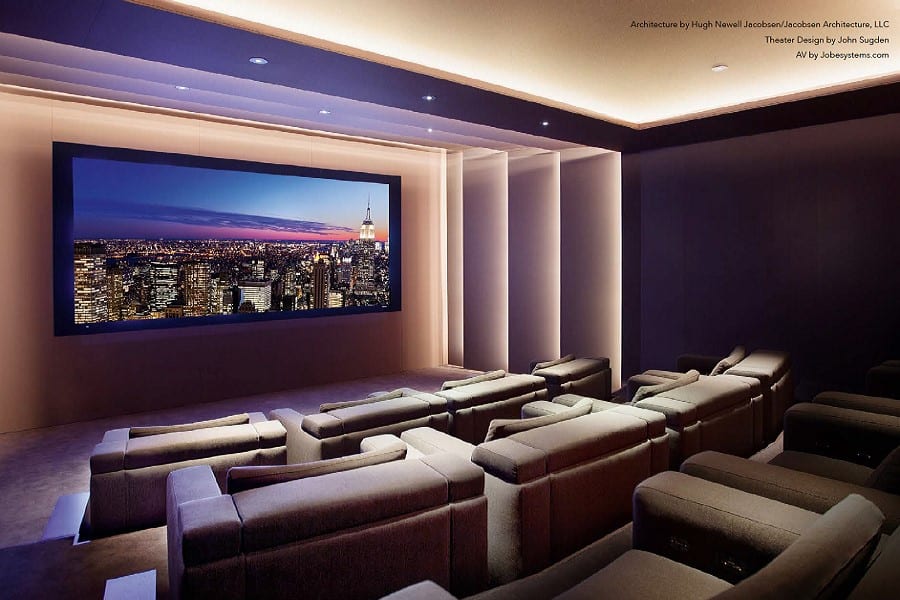This photograph captures an elegant private home theater room with an inviting and sophisticated ambiance. Dominating the right side of the image is a very wide, large-screen TV, currently displaying a city skyline at sunset with tall skyscrapers lit up against streaks of pink, blue, and purple hues in the sky. The room features several plush, oversized beige sofas with wide arms, arranged in a staggered formation from the bottom left toward the center and the middle-right of the image, suggesting maximum comfort for viewers. The ceiling and walls of the theater room showcase a gradient of colors, transitioning from light purple near the screen to a darker purple and eventually beige towards the edges. Discreet architectural credits are visible at the top right corner of the image, including "Architecture by Hugh Newell Jacobson, Jacobson Architecture LLC" and "Theater Design by John Sugden." Despite the luxurious comfort of the seating, there are no ottomans visible, indicating that viewers likely nestle directly into the generously proportioned chairs.